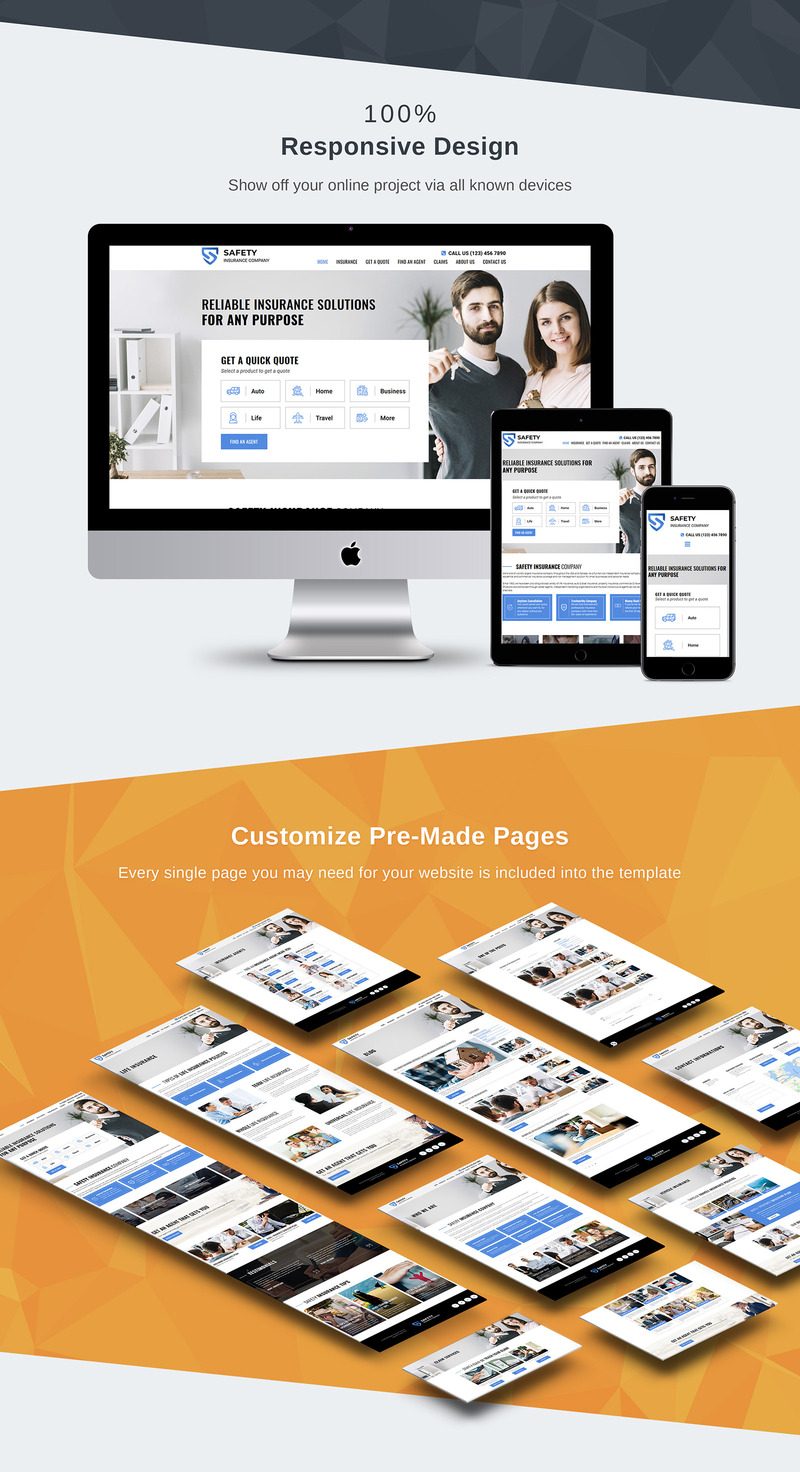**Caption:**

This mobile-sized advertisement showcases a sleek, modern design that highlights the responsiveness and versatility of a web template. At the top, a dark gray slanted bar introduces the composition, seamlessly transitioning into a larger light gray section. This predominant area features an Apple computer monitor displaying a vibrant image of a couple alongside a dynamic webpage. In front of the monitor, a tablet and a phone present distinct versions of the same webpage, emphasizing the theme of adaptive design. Bold text at the top proclaims "100% Responsive Design," with a compelling tagline beneath: "Show off your online project via all known devices."

The lower half of the ad is striking with an orange background contrasting the white text that reads: "Customize Pre-made Pages." This section elaborates, "Every single page you may need for your website is included in the template." A collage of various webpage portions, arranged in different colors and styles, provides a visual testament to the diversity and customizability of the template offerings. This ad effectively conveys the message that the template can meet a multitude of design needs across various devices.